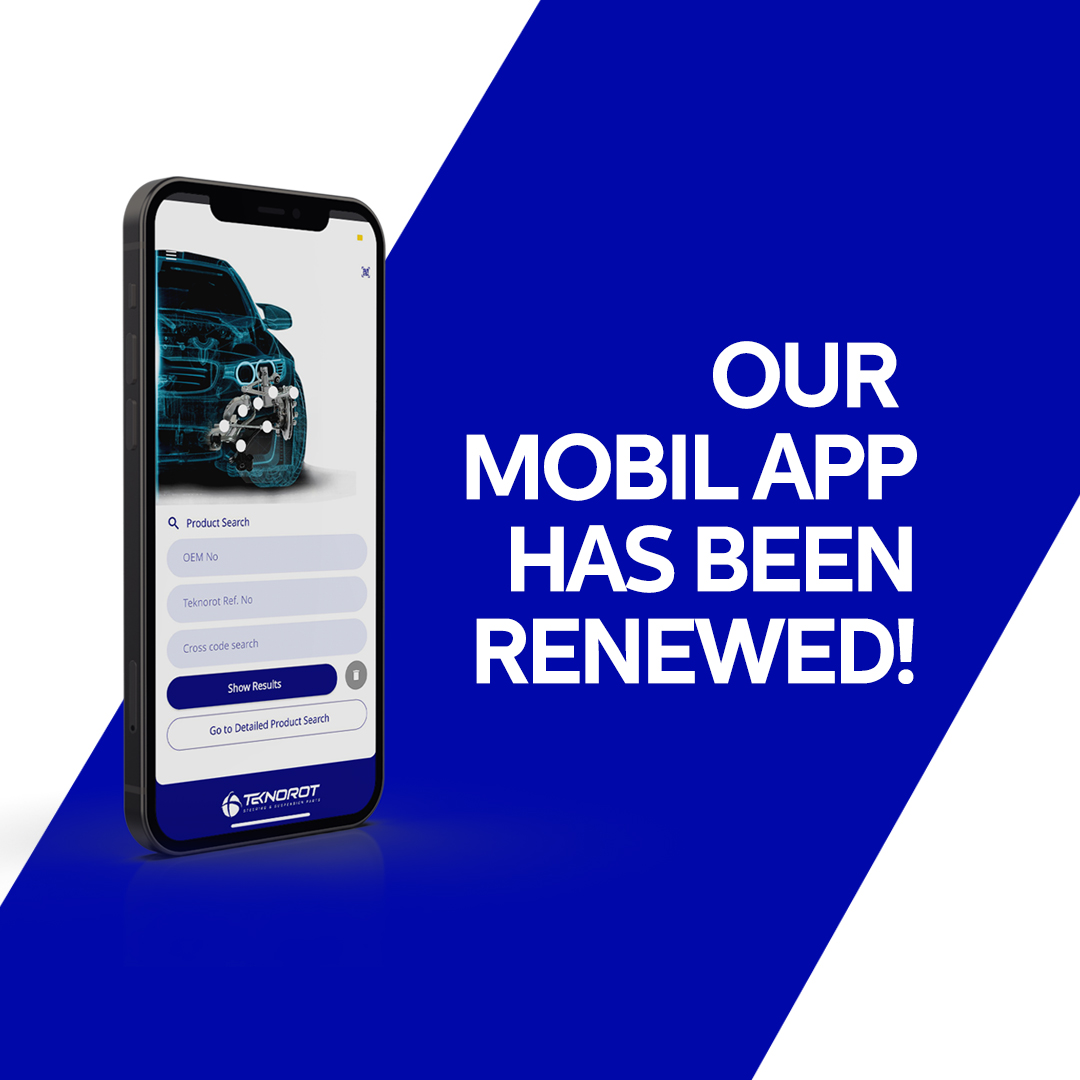The image features a detailed illustration showcasing new functionalities of a mobile app. On the left side, a cell phone outlined in black stands prominently against a white background. Adjacent to the phone, there is a vibrant depiction of a vehicle, presented with an electric aesthetic. Numerous lines resembling electric wires traverse the vehicle, uniquely colored in bright blue to highlight various features.

At the front wheel of the vehicle, eight distinct white circles are displayed, accompanied by a small magnifying glass icon labeled "Product Search." Below this section are three interactive blue circles, each clickable to reveal additional information. Another dark blue circle below, labeled "Cross Code Search," invites further exploration.

At the very bottom, a dark blue circle reads "Show Results," followed by a white circle instructing users to "Go to Detailed Product Screen." A blue line and an additional white circle complete the bottom section of the illustration.

On the right side of the image, bold white text announces, "Our mobile app has been renewed!" The text is set atop a long diagonal rectangle filled with a bright blue color, making the announcement stand out prominently.